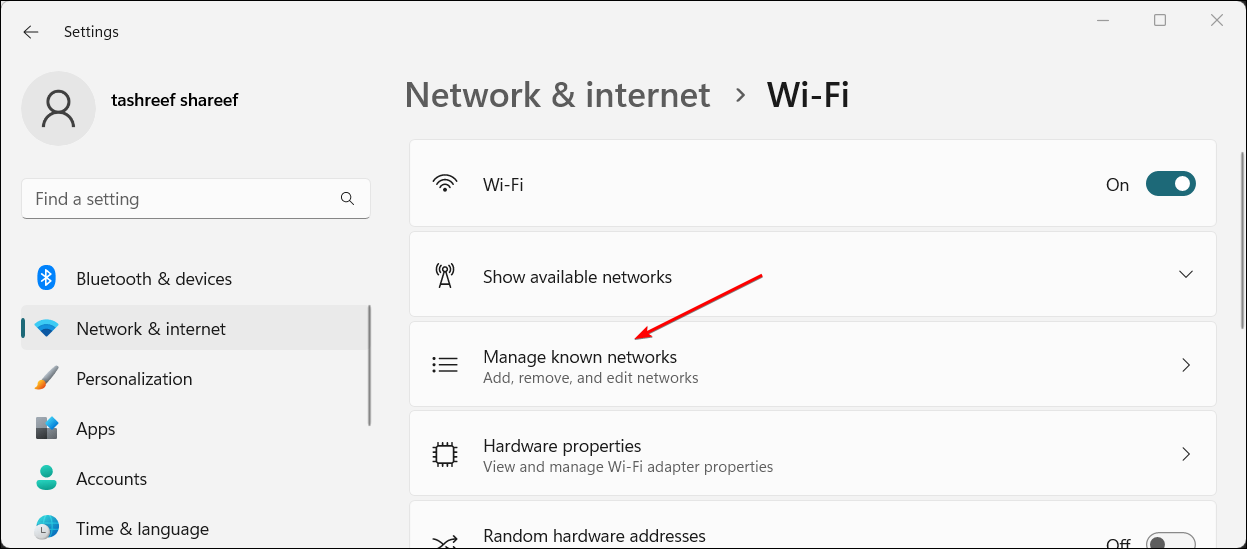The image depicts a section of a settings page from what appears to be a digital interface. In the top left corner, there is a "Settings" label with an arrow pointing to the left, suggesting a navigation option to go back. Beneath the label, there is a user icon accompanied by the name "Tashreef Sharif."

Below the user information, there is a searchable rectangle with a magnifying glass icon and the placeholder text "Find a setting." Further down, there are several menu options listed in order: Bluetooth & Devices, Network & Internet, Personalization, Apps, Accounts, Time & Language.

At the top center, the page prominently displays the section title "Network & Internet" in large letters, with an arrow pointing to the Wi-Fi section. Directly below, there is a Wi-Fi heading accompanied by a toggle button indicating that Wi-Fi is turned on. Following this, there are several interactive options: "Show available networks," "Manage known networks," and “Add, remove and edit networks.” A red arrow is distinctly drawn pointing towards the "Manage known networks" option.

Below these options, there is a section titled "Hardware problems," followed by "Random hardware addresses." Next to the "Random hardware addresses" label, there is another toggle button which is switched to off.